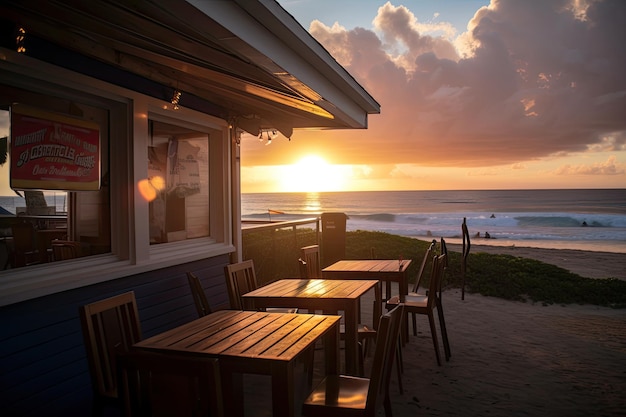The image portrays a picturesque beachside scene at sunset, capturing the serene beauty of nature. In the foreground, there's a restaurant with large windows, flanked by a scattering of wooden tables and chairs, each table accompanied by two chairs of the same design, neatly pushed in. The restaurant looks calm and mostly empty, with a red sign above bearing unreadable yellow and blue text. Surrounding the restaurant is sand, with a small green patch of grass leading toward the beach. The sky is a stunning blend of pink, purple, yellow, and white hues, reflecting the magic of the setting sun. The clear day, dotted with masses of clouds, enhances the tranquility of the scene. Along the shore, people can be seen enjoying the water, swimming, and surfing, while one figure walks in the distance. There's also a trash can near the restaurant, underscoring the more mundane details of the scene. This idyllic snapshot seems to be taken by someone with a keen appreciation for natural beauty.